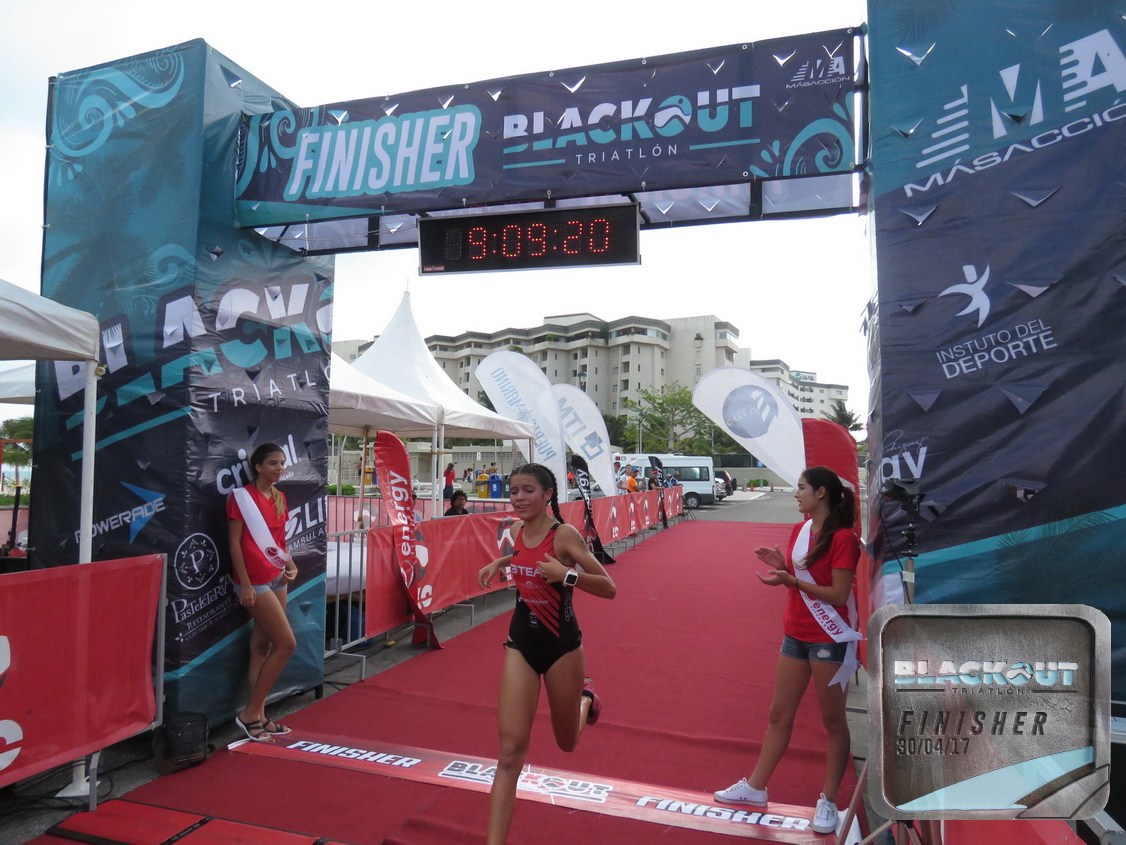In this wide rectangular photograph, we capture the energetic scene of a finish line at a running track, meticulously set up for a triathlon event. The track itself is covered with a striking red carpet, prominently marking the finish area with a sticker that reads "Finisher." Above, an archway displays the event logo "Blackout Triathlon Finisher," and a digital clock hanging from the archway shows the time, 09:09:20 in bright orange lights.

At the bottom center of the image, a woman with braids, wearing a red and black leotard with white lettering, sprints past the finish line. She has light brown skin and a white smartwatch on her wrist. Her left leg is firmly on the ground while her right leg, clad in a running shoe, is bent behind her in mid-stride. Her forward momentum and determined expression embody the spirit of the race.

Flanking the finish line are two women dressed in red tops and jean shorts, each sporting a white sash across their chest. Their hair is tied back in ponytails as they stand in supportive roles at the culmination of the race.

In the background, beyond a metal fence, white tents are visible, likely housing race amenities or spectators. Further back, vehicles and a large multi-story apartment complex can be seen, adding depth to the urban setting of the event. This comprehensive scene encapsulates both the intensity and celebration at the finish line of a triathlon.